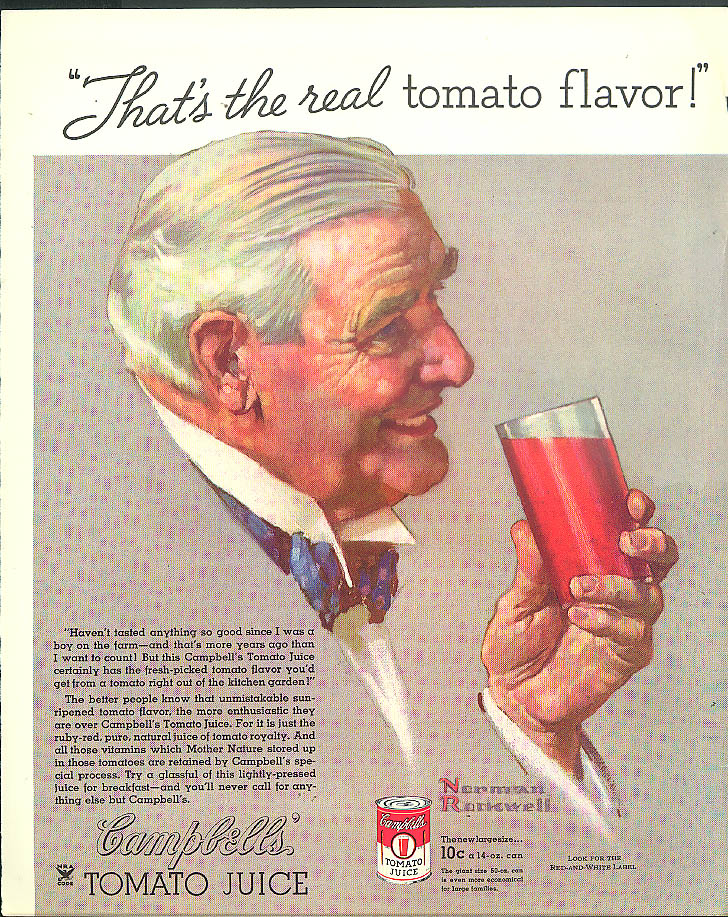This advertisement for Campbell's Tomato Juice features a classic, old-fashioned design evocative of the mid-20th century. Dominating the center is a detailed illustration of Norman Rockwell, depicted as an elderly man with grayish-white hair, expressive wrinkles, and a rosy complexion. Rockwell is smiling warmly, dressed in a white collared shirt paired with a blue polka-dotted bowtie. His right hand is elegantly holding a nearly full glass of tomato juice, poised as if he’s about to take a sip. 

Above Rockwell's head in a white border, the ad proclaims in cursive black text, "That's the real tomato flavor!" Below his image, there's a heartfelt testimonial in black text, which reads, “Haven't tasted anything so good since I was a boy on the farm.” At the bottom left, the text “Campbell's Tomato Juice” is prominently displayed, while to the right, there’s a smaller illustration of a Campbell's Tomato Juice can, styled in the familiar red and white. Accompanying this is a note that details the price: “Large size 10 cents, 14 ounce can,” along with Norman Rockwell’s name. The background is a simple gray, which keeps the focus on Rockwell and the product.